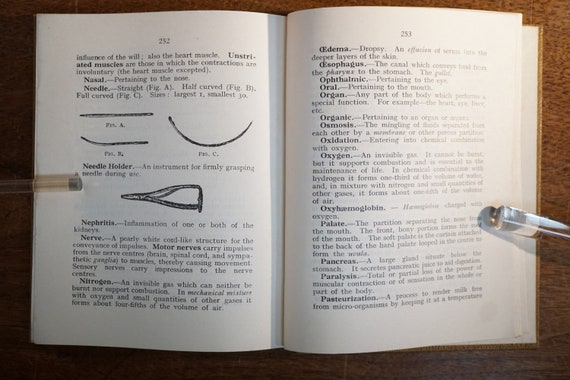The image depicts an open book, appearing to be a science or medical textbook, laid out on a dark wooden desk. The left-hand page is numbered 232 at the top, while the right-hand page is numbered 233. On the left page, there are six or seven lines of black text followed by a series of figures: one horizontal black line, another horizontal line that curves upward at the left, and a curved black line. Below these are two more lines of text and an additional figure, followed by more paragraphs of writing. The right-hand page resembles a glossary or dictionary, featuring 14 bolded words with their definitions. The words include medical terms such as "edema," "esophagus," "ophthalmology," "oral," "organ," "organic," "osmosis," "oxidation," "oxygen," and "oxyhemoglobin."

A transparent tube, possibly made of glass or plastic, is positioned on the left side, with a bit of it touching the left page. A similar tube is on the right side, partly visible and extending off the image just below the center. These tubes, or pen-like instruments, contain silver elements inside. Additionally, a hint of the book's back cover is visible to the right of the right-hand page. The detailed terminology and figures suggest that the book deals with anatomy, physiology, or medical procedures, emphasizing the focus on organs, nerves, and related medical terms.